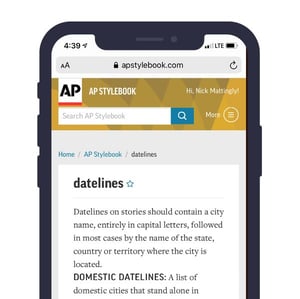This detailed caption captures the partial upper half of a smartphone screen displaying a vibrant photograph. The screen exhibits typical smartphone elements, such as the current time positioned at the top-left corner, and indicators for signal strength, LTE connectivity, and battery life at the top-right.

Prominently displayed is a text banner that reads "APStylebook.com." Below this, another banner states "AP Stylebook" with a greeting, "Hi, Nick [Last Name]." Immediately under this banner is a small search text box, encouraging direct inquiries. 

Further down, a navigation path is shown: "Home > AP Stylebook > Dateline," with the term "Dateline" highlighted. The accompanying text provides an explanation about datelines: 

"Datelines should contain a city name, entirely in capital letters, followed in many cases by the name of the state, country, or territory where the city is situated. Datelines on domestic stories may also include a list of cities that stand alone."

The final line under this text, written in bold black letters, emphasizes "DATELINES" with an asterisk. It includes the guideline's initial portion, explaining how city names in datelines should be used and formatted in stories. The text cuts off as it begins a section on domestic datelines.